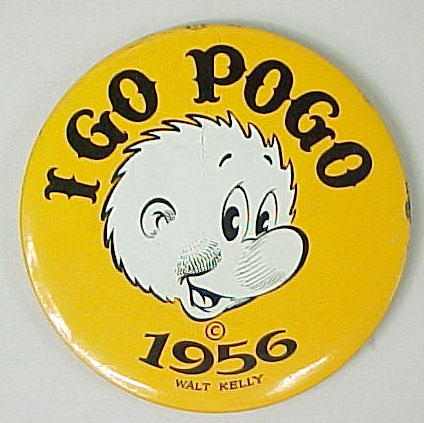The image features a round, mustard-green pin from 1956, created by Walt Kelly. The pin displays the phrase "I go Pogo" in bold, black, all-capital letters at the top. Below the text, there is a black and white illustration of a whimsical, furry character with spiky hair around its head. The character has a large nose, a wide smile with an open mouth, and one visible ear. The design is distinctive with its raised eyebrows and prominent facial features. Beneath the drawing, the pin is marked with a copyright symbol and the inscription "1956 Walt Kelly." The pin rests on a grey background, making it stand out clearly.